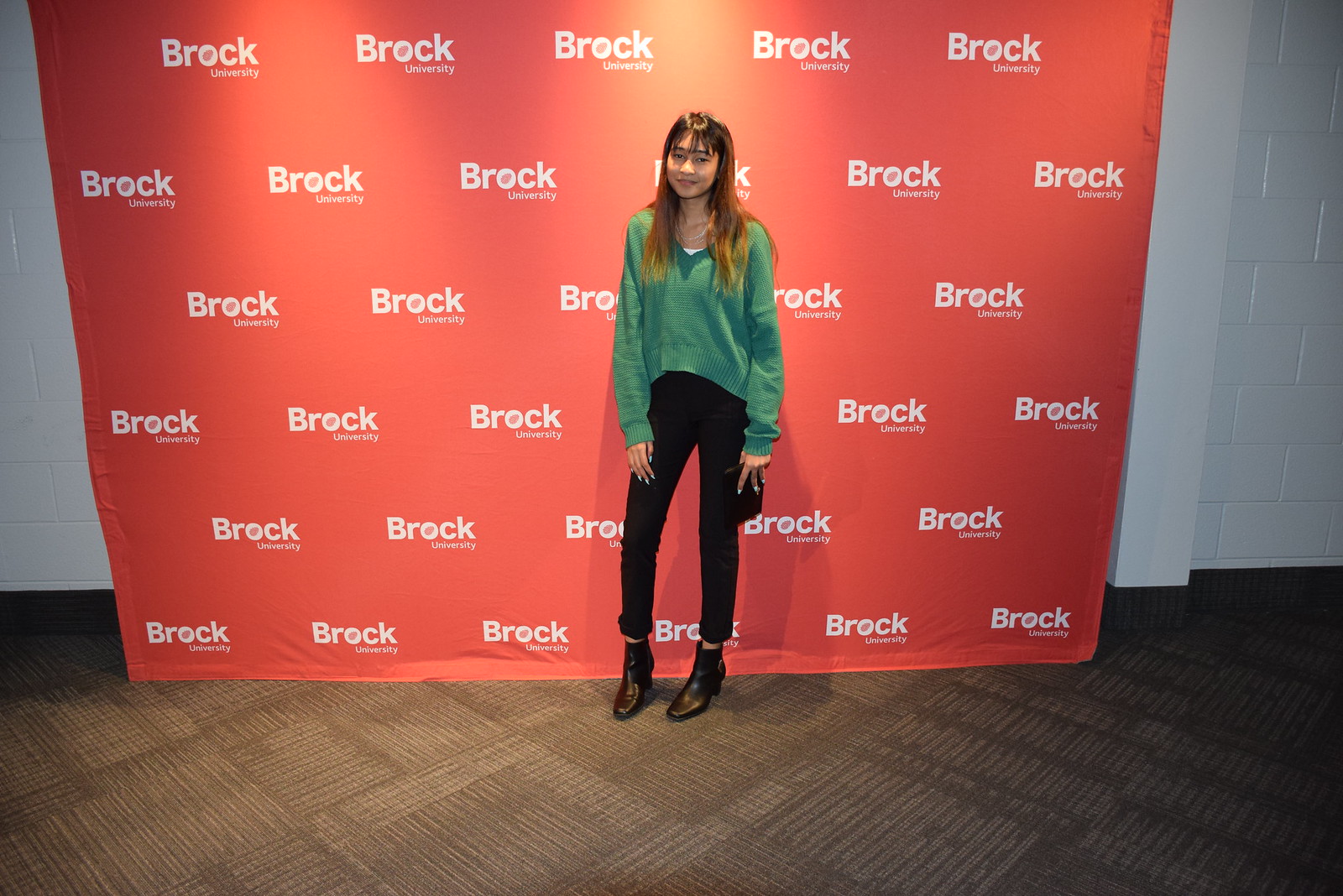The photo captures a young woman standing in front of a repeated "Brock University" backdrop, which appears to be designed for photo opportunities at an event. The backdrop is predominantly red with white text and is framed by a white brick wall on either side. She stands on a brown carpet composed of squared segments. The woman is wearing a long-sleeve green sweater over a white undershirt, black skinny pants that end slightly above her ankles, and small black boots. She holds a black clutch purse in her left hand, showcasing her teal-colored fingernails. Her long brown hair, with short bangs, extends to her chest and features blonde highlights at the tips. She also wears a necklace and has distinct dark eyebrows. Her appearance may suggest a mixed ethnicity, potentially Asian or Mexican.